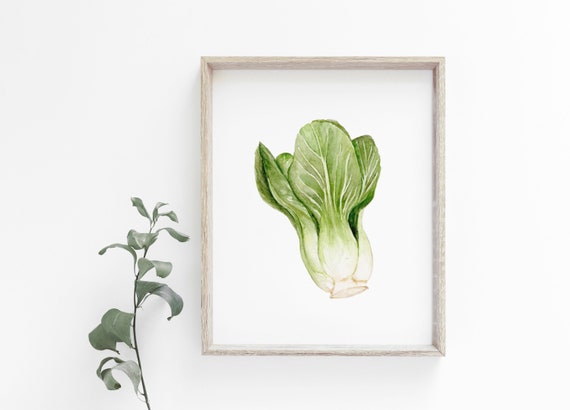The image is a detailed watercolor painting of a green leafy vegetable, likely bok choy, housed in a grayish wooden frame that features the natural texture of wood. This deep and somewhat shadow-box-like frame encloses the artwork, with the picture surface set below the edge of the frame, creating a sense of depth. The vegetable is depicted with white veining and a base where the leaves are attached, transitioning to rich green leaves that fan out in a circular pattern from the bottom. The background of the painting is white, emphasizing the minimalistic and organic feel of the image. Adjacent to the framed painting, on the left side, is a small, minimalistic plant with a long stem and leaves that are dispersed primarily at the bottom and top, complementing the color and style of the watercolor painting. This entire setup is mounted against a white wall, enhancing the serene and natural aesthetic of the composition.